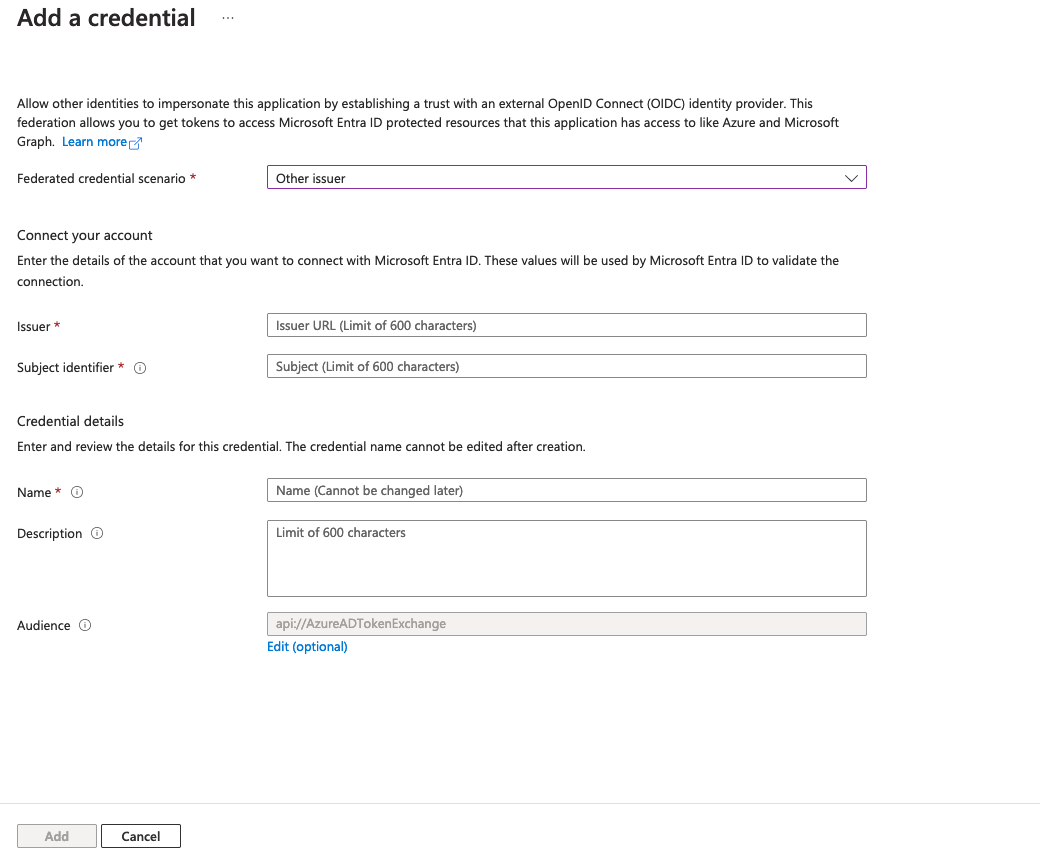The image showcases a form related to federated credentials within the Microsoft Entra ID system. The form enables users to allow other identities to impersonate the application using OpenID Connect (OIDC) and other providers, thereby granting access to Azure and Microsoft services. It features fields for entering the credential name, description, and issuer URL, which are required but currently empty. There's also a section for specifying the audience, with options such as 'API' and 'Azure AD' for token exchange. On the bottom left-hand side, there are 'Add' and 'Cancel' buttons, with the 'Add' button grayed out while the 'Cancel' button is black and bold. Essentially, this form appears to facilitate adding another user or identity for federated access within the Microsoft Entra ID framework.